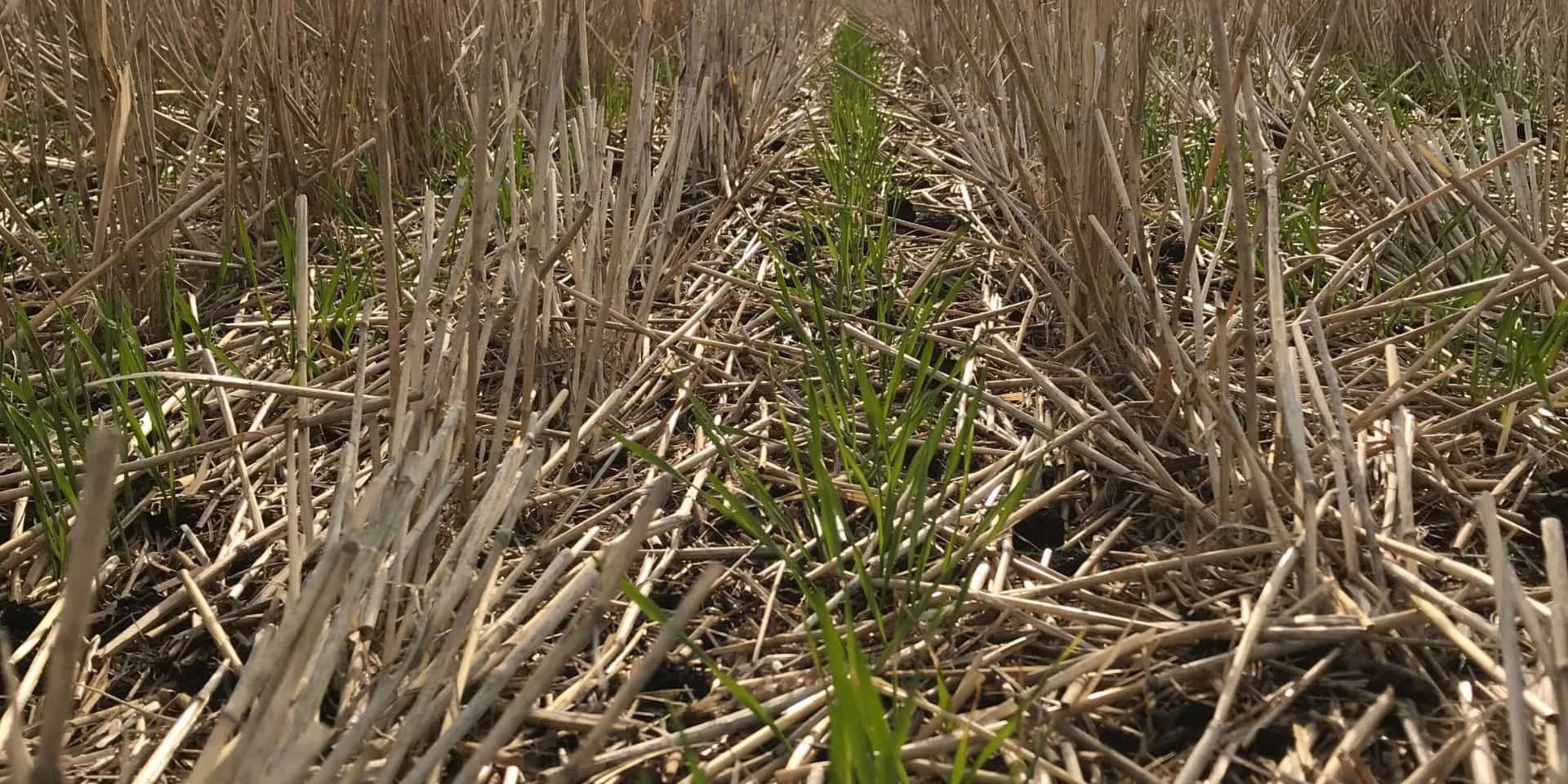The image captures the aftermath of a recent harvest in a vast field, stretching from the foreground far into the horizon. The photograph is taken in the afternoon, casting a mellow light over the landscape. Rows of tan, dried stalks of plants, all uniformly cut and partially bent as if compressed by machinery, dominate the scene. Between each row runs a trail of vibrant green grass, creating a striking contrast with the desolate rows of straw-like material. Scattered throughout, there are patches where the stems appear darker brown and less dried out. To the sides of the central green trails, the ground is interspersed with more greenery and tall grass, adding to the texture and depth of the image. The entire composition is a testament to the meticulous order of harvesting, blended with the remnants of life asserting themselves through the patches of green.